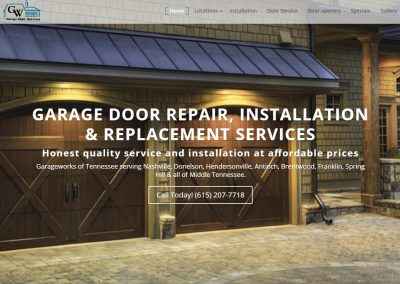A small promotional image for a garage door repair website featuring essential information and visual elements. Prominently in the center, bold white text reads "Garage Door Repair, Installation, and Replacement Services," indicating the primary services offered. The background showcases a pair of large, wooden garage doors situated in a white driveway, framed by a white brick wall adorned with lights. Above, a distinctive blue roof adds a touch of contrast to the scene. 

In the top left corner, the company logo is visible, consisting of black letters "GW" surrounded by a blue outline resembling a house, though the accompanying small text appears slightly blurry. On the top right, a gray box houses navigational links for the website, with the active "home" link highlighted in white amidst other gray-highlighted links.

Below the central text, additional information about the company's services is provided. A white box with transparent background displays "Call Today" along with the phone number 615-207-7718, encouraging immediate contact for service inquiries.